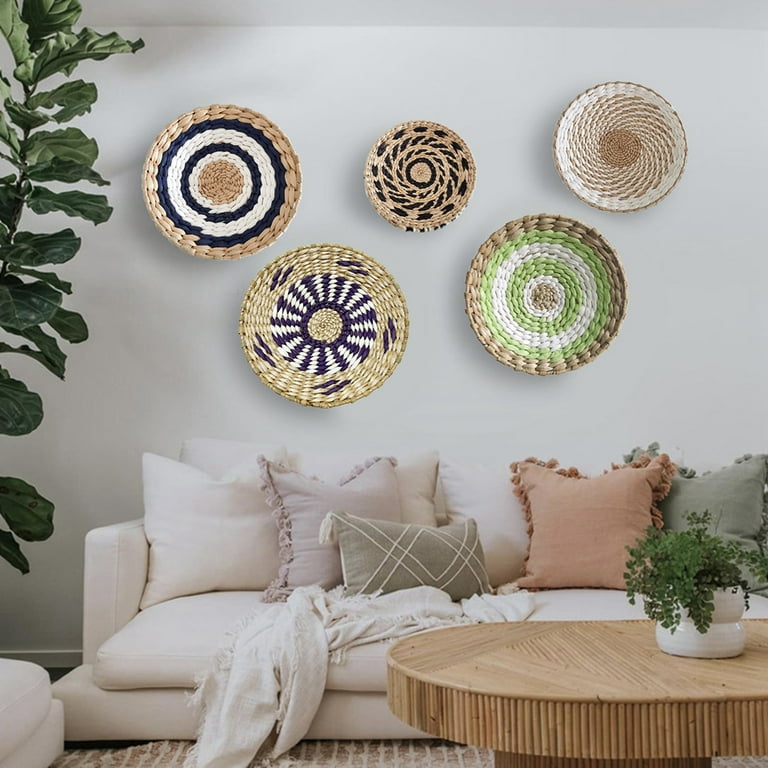The image showcases a modern living room with an off-white wall adorned by five decorative woven plates, each with unique designs and color patterns. Starting from the top left, one plate features black and white rings with a brown center and outer edge. The center plate is predominantly brown with black dots encircling it. The upper right plate is primarily white with a brown center and looping brown patterns around it. The lower left plate has brown, black, and white patterns resembling an eyeball shape. The lower right plate alternates between green and white circles with a central brown area.

Below the woven plates, there is a beige, low-setting couch covered in linen that extends close to the floor. The couch's back is lined with various pillows in hues of beige, brown, reddish, and green, along with a thin linen throw blanket draped over it. In front of the couch, a low coffee table, made of thin pieces of inlaid wood, holds a small potted fern plant in a white pot. To the left of the scene, an indoor tree plant with large green leaves extends upwards, adding a vibrant touch to the room's natural and modern aesthetic. The overall decor emphasizes simplicity, sustainability, and a tranquil, environmentally-friendly atmosphere.